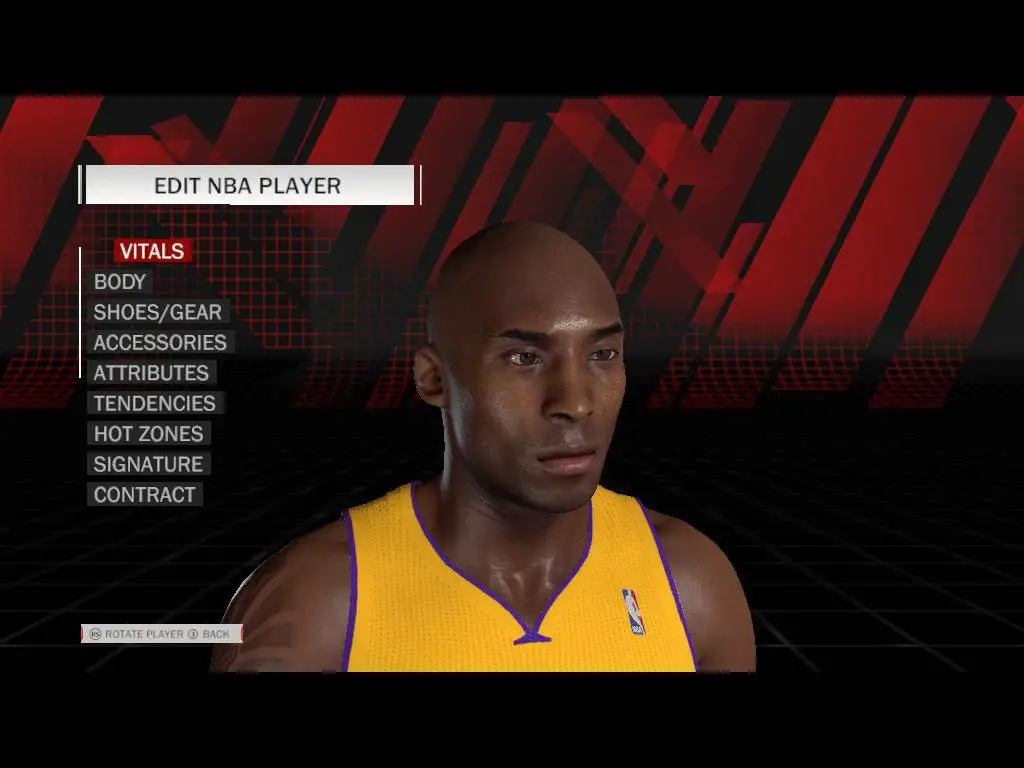The image depicts a character creation screen for an NBA video game. The background is predominantly black with a grid pattern of white lines forming squares. In the center, there is a visual of a video game character with the label "PS2B" in bold black and red text. A white bar just above the character reads "Edit NBA Player."

The player model is very detailed, with dark skin, a noticeably sweaty face, and clearly defined facial features, including a nose and mouth. The character is dressed in a yellow jersey with purple accents, reminiscent of a Los Angeles Lakers uniform, complete with the official NBA logo.

On the right side of the screen, there is a red rectangle with white text displaying the word "Vitals." Below this are categories listed in gray text: Body, Shoes, Accessories, Attributes, Tendencies, Hot Zones, Signature, and Contracts.

At the bottom of the screen, there are interface elements with options such as "Rotate Player" and "Back." The floor and background feature the same black tiling with white grid lines as the rest of the setting, creating a uniform visual theme. This screen is part of the process for customizing a player's appearance and attributes in the game.